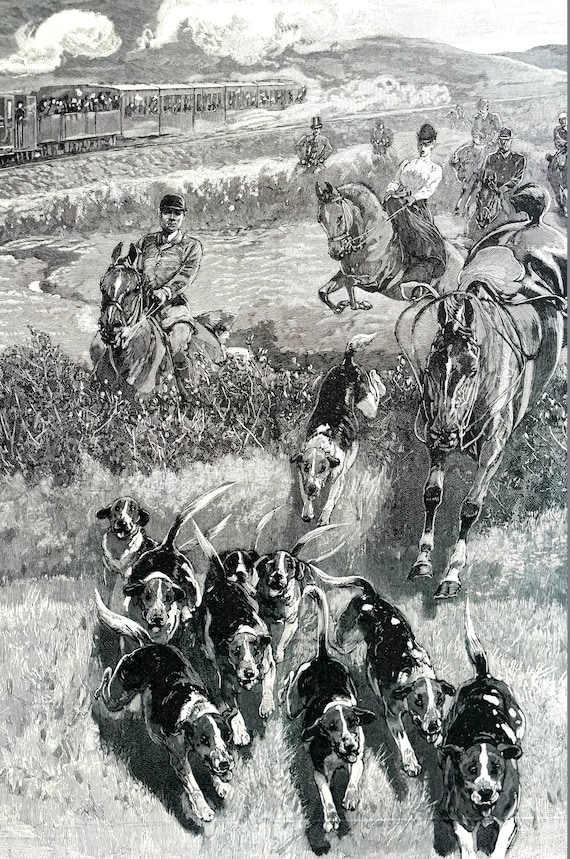The image is a black and white rendering of an old-fashioned fox hunt, probably a photograph of an original painting given its slightly cropped appearance marked by a grey line down the right-hand side. Central to the scene is a dynamic portrayal of a pack of small to medium-sized hunting dogs, distinguished by their black backs and white-striped faces, energetically running towards the viewer with their tails aloft. Just behind them, a group of riders can be seen on horseback, attired in period clothing with one female rider notably wearing a black dress and white top, riding side-saddle. Interestingly, one of the horses is unmounted, adding a sense of realistic action, possibly suggesting that a rider has fallen. The hunt appears to traverse through marshland, enhancing the traditional ambiance of an English countryside pursuit. In the top left corner, a railway track runs parallel to a hillside, upon which an old steam train chugs along, its passengers seemingly observing the hunt unfold below. The seamless integration of these elements evokes a vivid, historical scene reminiscent of an era long past, despite the absence of the artist's signature or a precise date.